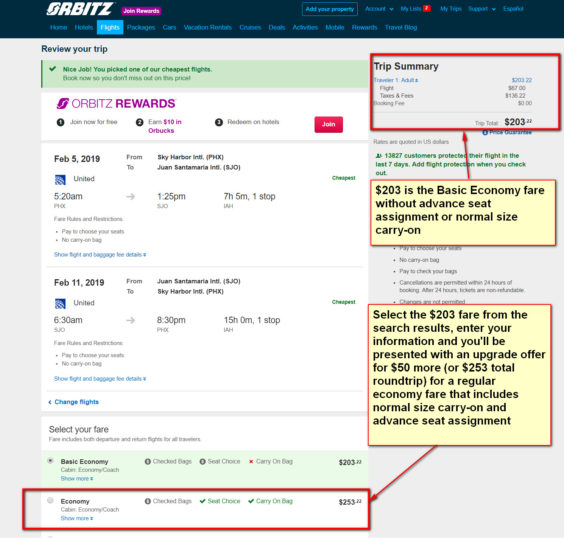The website depicted is Orbitz, identifiable by its dark blue navigation bar at the top. On the top left corner, the "Orbitz" logo is prominently displayed. Adjacent to the logo, there's a purple button labeled "Join Rewards." The main content of the page includes a section titled "Review Your Trips." Within this section is a light green bar featuring a checkmark icon and the message, "Nice job! You picked one of our cheapest flights. Book now so you don't miss out on the price."

On the right side of the page, there are several vertically stacked boxes, each outlined in red. The first box at the top is labeled "Trip Summary." Below this, an arrow indicates details about a fare option: "$203 is the basic economy fare without advance seat assignment or normal-size carry-on."

Another box underneath provides action steps: "Select the $203 airfare from the search results. In your information, you'll be presented with an upgrade offer for $50 more or $253 total round-trip for a regular economy fare that includes a normal-size carry-on and advance seat assignment."

At the bottom of this section, the final price is outlined in red, providing a clear and concise overview of the total cost.